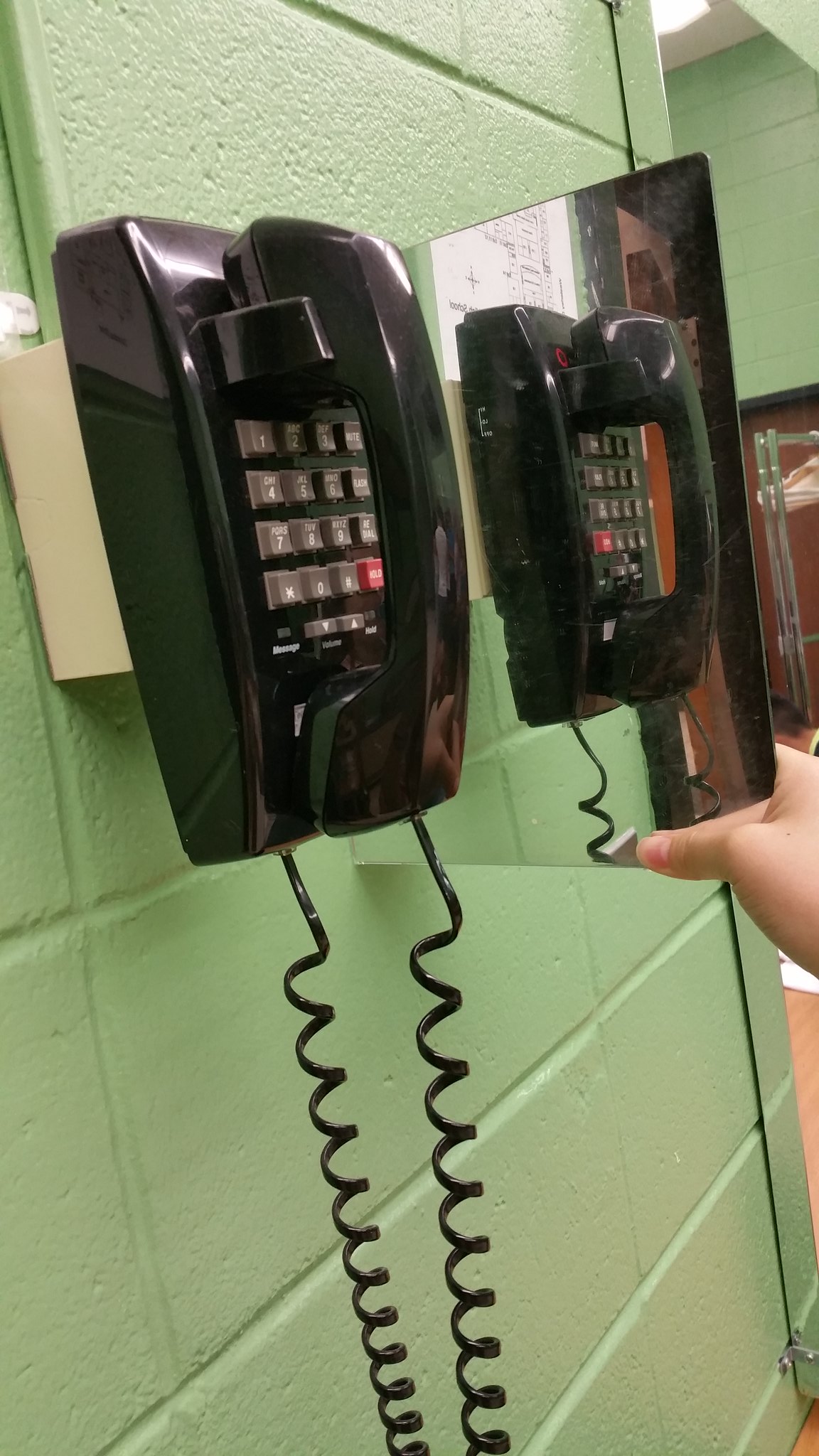The image showcases two vintage black telephones mounted on a green concrete block wall. Each phone features a long, black, spiral cord connecting the handset to the wall-mounted base. The keypads are composed of gray keys with white numbers and letters, arranged in a square layout, indicating numbers 1 through 9, 0, and special characters. A red button on each phone, presumably the hold button, stands out, along with volume control buttons for adjusting the sound. An indicator light on each phone likely signals new messages or active holds. In the scene, there's a hand holding a mirror, reflecting one of the telephones, and revealing additional reflections down the line. The setup hints at a public telephone or a shared communication space from a bygone era.